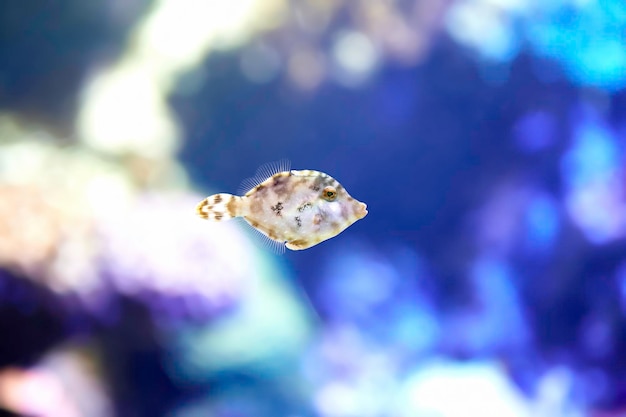This zoomed-in, square, color photograph features a very tiny fish as the focal point. The fish has a leaf-shaped body that is primarily white with patches of brown and gray spots. Particularly notable are the markings on the tip of its tail that resemble a smiley face in brown. The fish is depicted in profile, appearing as though it is swimming, and has tiny fins on its back and underneath its body, along with very small puckered lips. The blurred background encompasses shades of blue, possibly representing the inside of a fish tank or the ocean floor, with hints of coral and the sea. The background also features a marbleized, modern look with a mix of dark blue, light blue, white, and yellow hues.